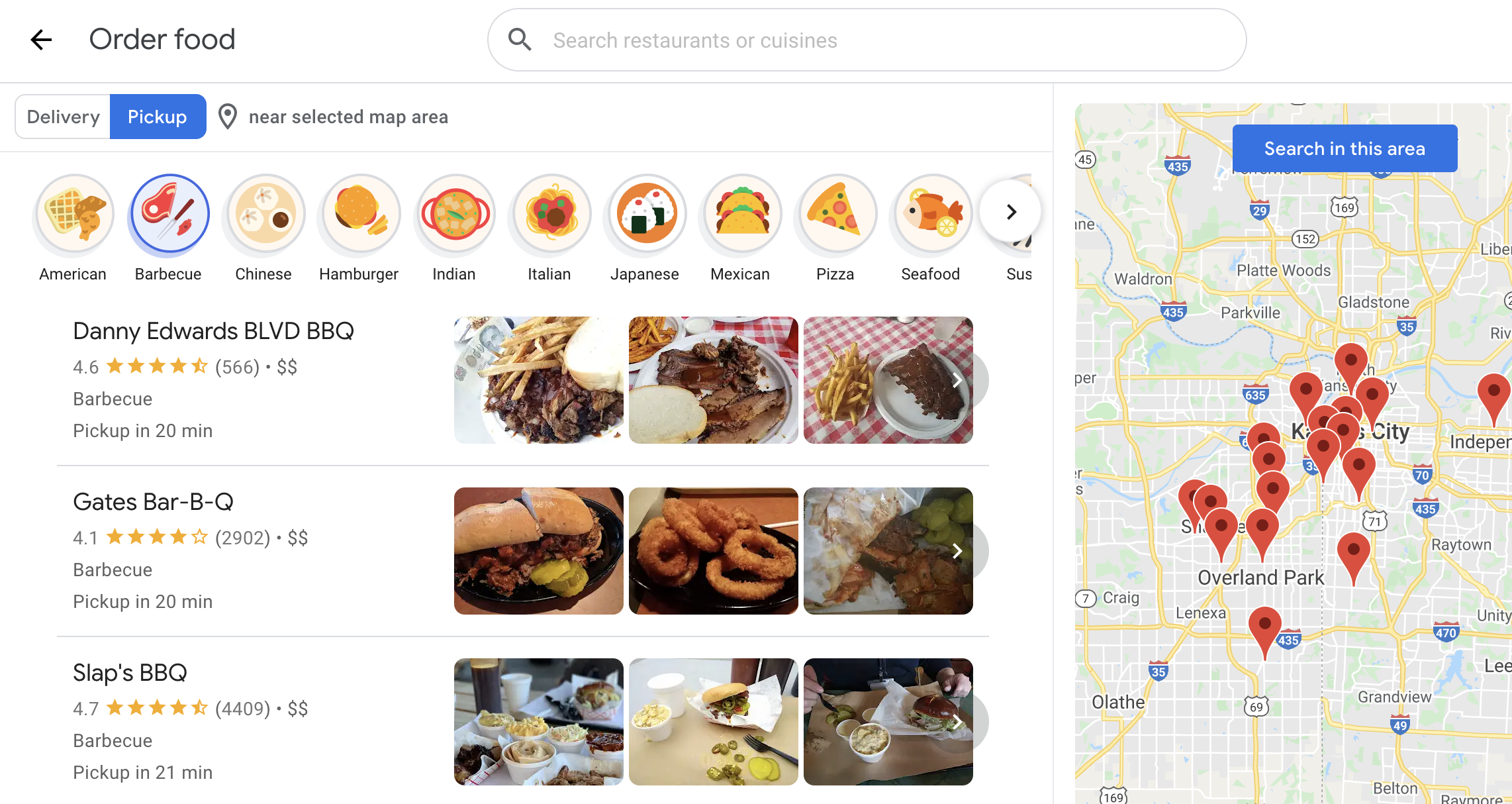On the food ordering website, the top section prominently displays a banner that reads "Order Food." Directly beneath this banner, there is a search bar where users can look up restaurants or specific cuisines. Just below the search bar are two options: "Delivery" and "Pick-Up," with the "Pick-Up" option highlighted in blue. A location icon below these options indicates that the search results pertain to the area near the selected map location.

Following this, the website allows users to filter their choices by cuisine, featuring categories such as American, BBQ, Chinese, Hamburger, Indian, Italian, Japanese, Mexican, Pizza, and Seafood. Each category is accompanied by a representative image; for instance, the Mexican cuisine is depicted with a picture of tacos, while the Japanese cuisine interestingly features an image of Hungarian food.

Among the search results, the first listing is "Danny Edwards BLVD BBQ," which boasts 566 reviews and a rating of 4.6 stars. The webpage mentions that pick-up is available in 20 minutes, and includes images of dishes like briskets and fries.

The next restaurant is "Gates BBQ," which has amassed 2902 reviews and holds a 4.1-star rating. Accompanying photos show items such as onion rings and a BBQ sandwich.

The third result features "Slaps BBQ," which stands out with 4409 reviews and an impressive 4.7-star rating. As with the other listings, images of their BBQ offerings are provided, offering a visual glimpse of the delectable options available.